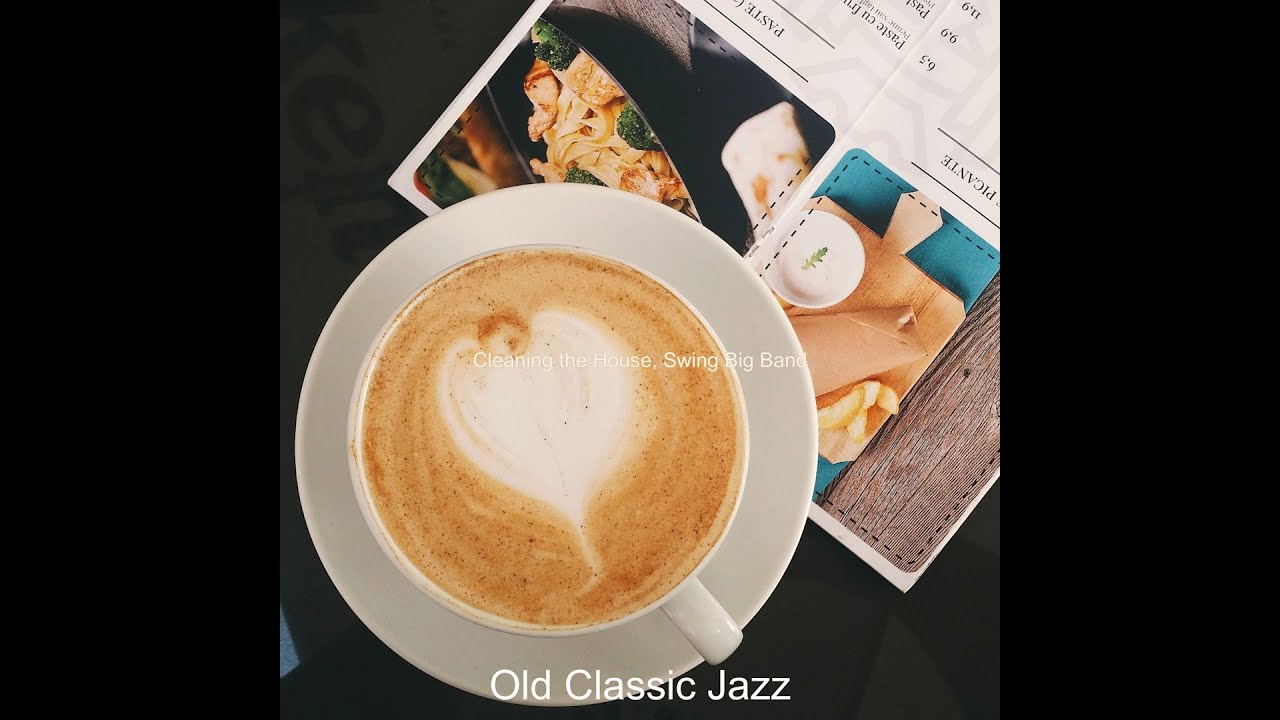In a top-down, landscape-oriented, square-format color photograph set against a black background, a meticulously arranged scene captures a white coffee cup on a matching saucer. The coffee, adorned with a frothy heart in the center, emits a warm, inviting brown hue. Superimposed across the cup in white text, it reads, "Cleaning the house, swing big band." At the bottom of the photograph, more white text states, "Old classic jazz." 

Partially tucked under the right side of the saucer is a diagonal clipping of a restaurant menu, showcasing images of a black dish filled with fried food and another dish possibly containing macaroni or pasta. The visible, upside-down text on the menu includes "P-A-S-T-L-E" and "P-I-C-A-N-T-E," sectioned off with black lines above and below. This detailed composition, set on a restaurant tabletop, combines elements of photographic representationalism and realism, enhanced by the surrounding black columns framing the image.